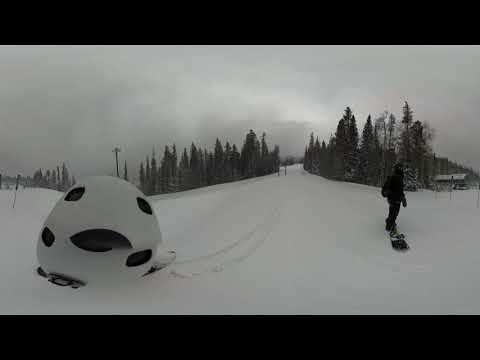The image captures a snowy, overcast winter day, likely in a ski area. The sky is almost as white as the snow-covered ground, with only a few darker gray patches indicating heavy clouds. In the foreground on the lower left, there is a peculiar, partially obscured object that looks somewhat like a distorted helmet. To the right, a snowboarder dressed in black clothes and goggles is gliding towards a clearing between two groups of snow-dusted evergreens. A row of trees, frosted with snow, stretches down the center of the image, flanked by another copse of trees to the far left. On the far right, a distant building stands against a backdrop of a hilly terrain. The entire scene is framed by a thick black border at both the top and bottom.